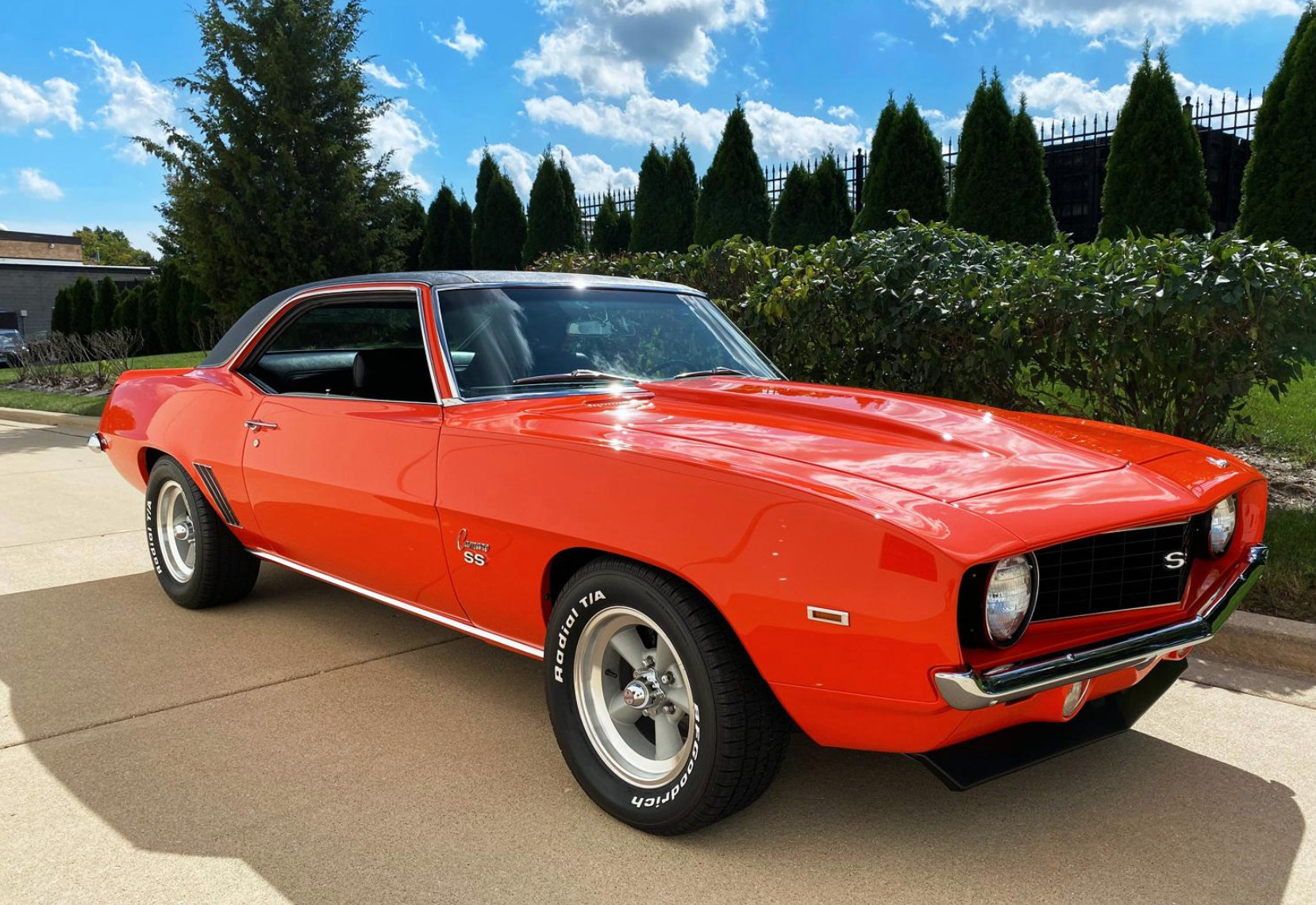An eye-catching photograph features a pristine, bright orange classic muscle car reminiscent of a late 60s model, possibly a Camaro. The car, gleaming with shiny red paint and a striking black hood, has a two-door design and is equipped with black wheels sporting silver rims, identified as BF Goodrich Radial T/A tires. The vehicle proudly displays an 'S' on its grill and boasts a black leather interior. With its convertible top up, the car appears brand new, as even the tires look completely unused. It sits parked in a long residential driveway, which is bordered by manicured shrubs and a tall gate with spikes. The background showcases a sprawling lawn, elaborate landscaping with manicured trees, and a large house under clear skies with sparse clouds. EdgeInsets such as the neatly designed surroundings and the luxurious setting complete the picturesque scene.